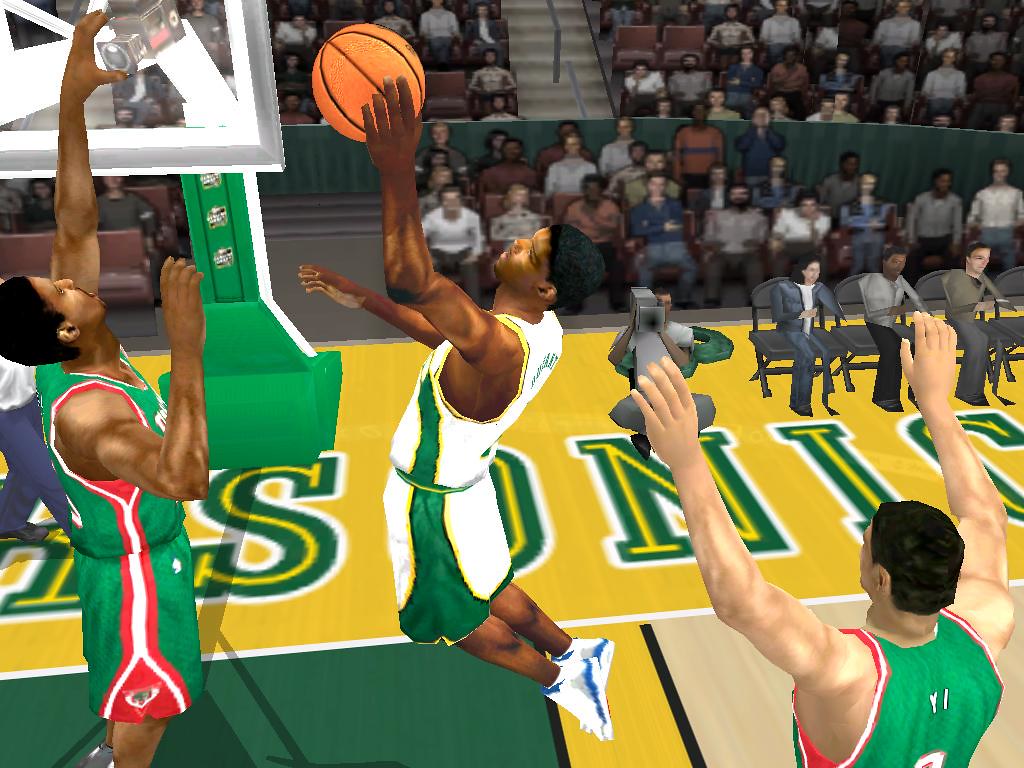In this screenshot from a video game, a basketball player poised for action is captured mid-motion, on the verge of executing either a layup or a slam dunk. The court is occupied by two teams, identifiable by their uniforms: one team clad in white jerseys and the other in green. In the background, behind the basket, a crowd is visible, though their faces are rendered indistinctly, appearing blurred and polygonal, which adds a surreal and somewhat peculiar element to the scene.